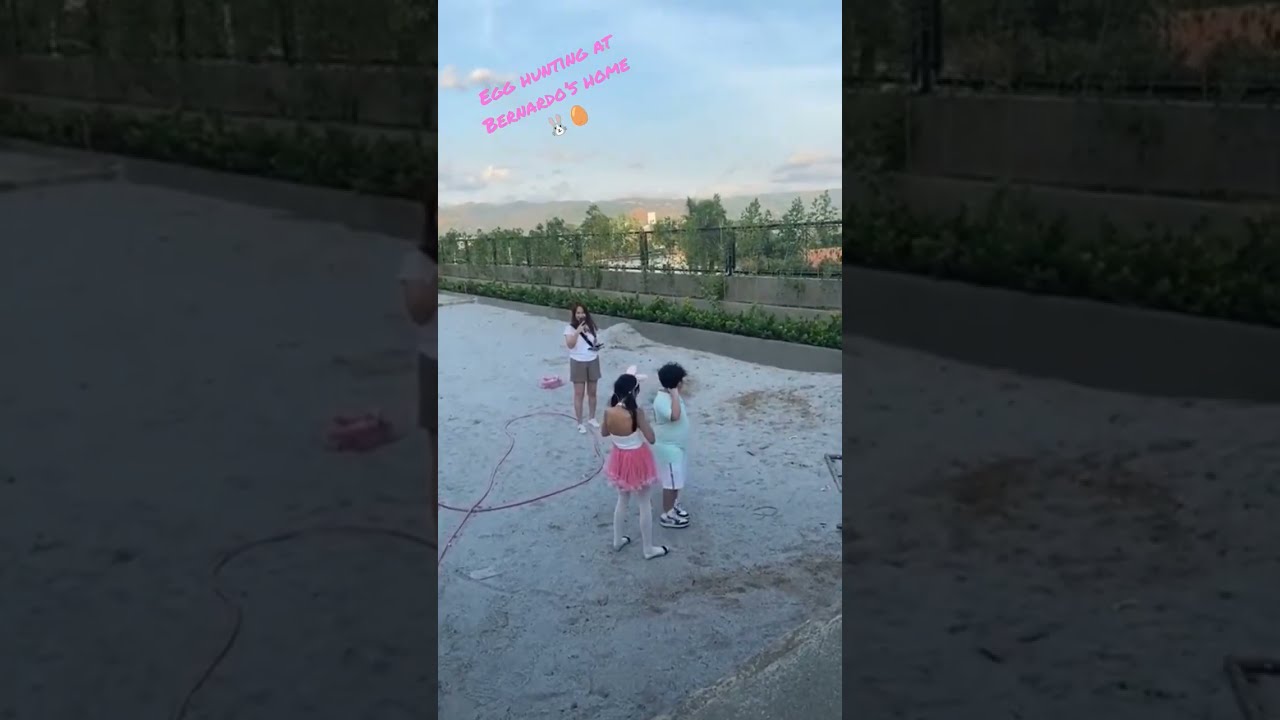In this vibrant outdoor setting, a group of children are on an Easter egg hunt, captured in a lively photograph. The scene unfolds on a stone ground, appearing like smooth, light-colored sand, with a nearby cement wall lined with lush green bushes and a taller mesh fence adorned with vines. The background features distant trees and a partly cloudy sky, indicating it's midday around Easter, as highlighted by the caption "egg hunting at Fernando's home" in the top left corner.

At the center of the image, two children and a woman are actively engaged. A young girl stands out in a pink tutu-like skirt, white top, white tights, and black sandals, topped with bunny ears, adding a festive touch. Beside her is a boy in shorts and a light teal shirt, embodying the playful spirit of the hunt. The woman, perhaps their guardian, holds up a phone, capturing the moment or recording a video. The joyous ambiance is reflected in the vivid colors of their attire and surroundings, including shades of light blue, white, gray, pink, yellow, black, and green, all contributing to the lively Easter celebration.